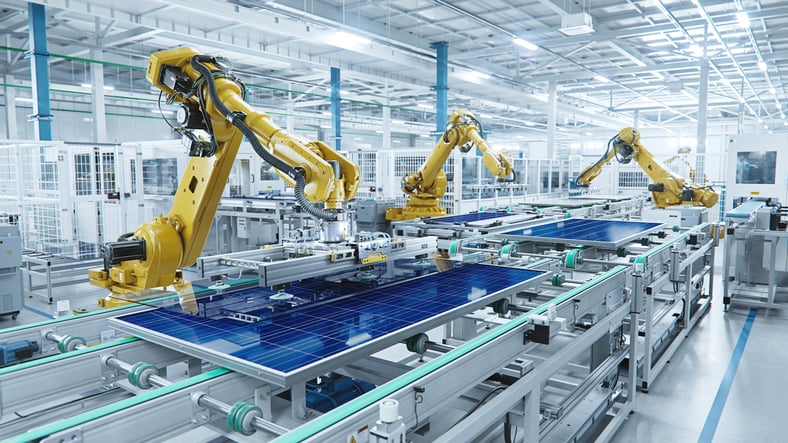The image showcases shiny, yellow pieces of equipment prominently featured in the foreground. These yellow components extend over a series of blue panels. White piping or tubing is visible on the ceiling of the image, indicating its function in an open and interconnected system. A notable feature includes a yellow arm or arrow, as well as a white box with a silver outline situated at the top of the image. The background elements and annotations suggest a separation of file names from vendor information, enhancing organizational clarity.